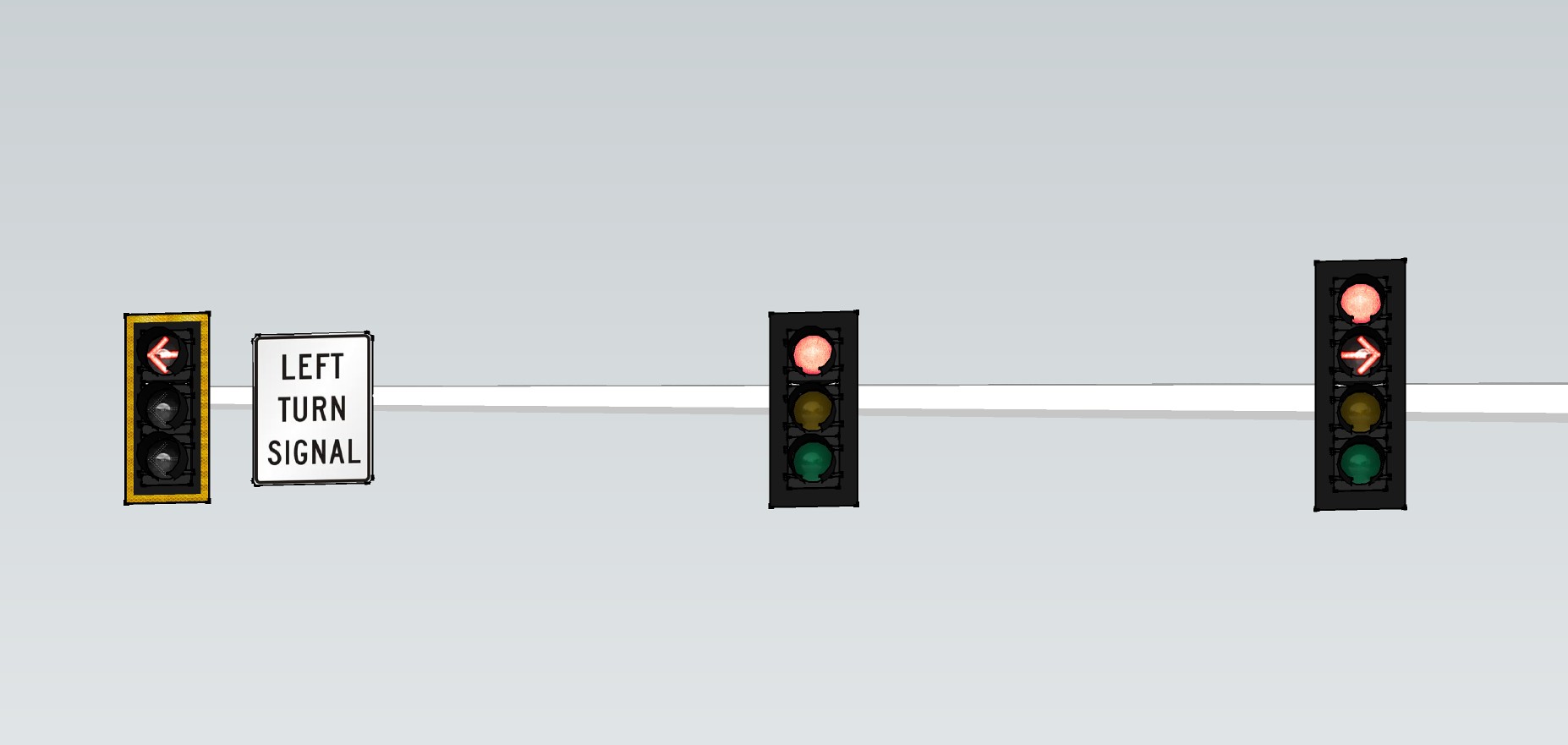The image is a digital rendering resembling an illustration from a driver's instruction manual. It depicts a section of an intersection with three traffic lights affixed to a single metal arm extending horizontally over what appears to be a street. The background features a muted, grayish-blue sky.

Starting from the left, the first traffic light is positioned furthest left, showing a red left-turn arrow that is currently illuminated. Adjacent to this light is a black sign with bold white letters reading "Left Turn Signal." 

In the middle of the arm, there is a standard three-light traffic signal. The top bulb, a red light, is illuminated, while the yellow and green bulbs beneath it are unlit.

On the far right, the third traffic light is more complex with four sections. The top light is solid red and lit, followed by a red right-turn arrow that is also illuminated. Below these are unlit yellow and green lights.

This detailed array of traffic signals provides clear indications for drivers, enforcing different rules for turning and stopping at this particular intersection.